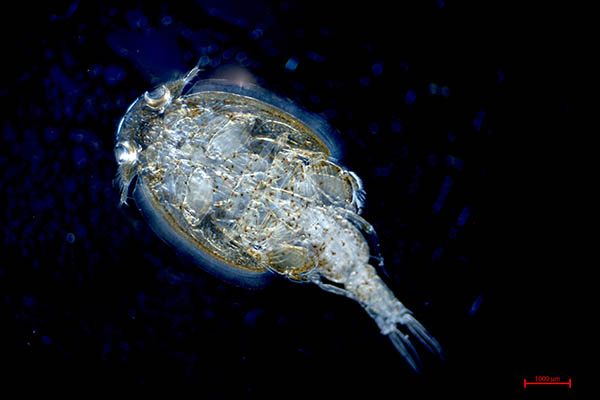This close-up, x-ray-type image reveals a small, transparent sea creature or plankton, occupying the center of the frame. The photograph, in landscape orientation and set against a black backdrop scattered with small blue dots, highlights the intricate details of this bizarre-looking organism. The creature's oval-shaped body, which is partially transparent, showcases colors ranging from gold, white, gray, to blue. It features a relatively thin tail with fins, adorned with strands at its end. Prominent on its body are two large, bulging eyes. Surrounding the edge of its body is a thin, shell-like structure. In the bottom right corner of the image, a red scale measuring 1000, possibly micrometers, indicates the minute size of the creature.